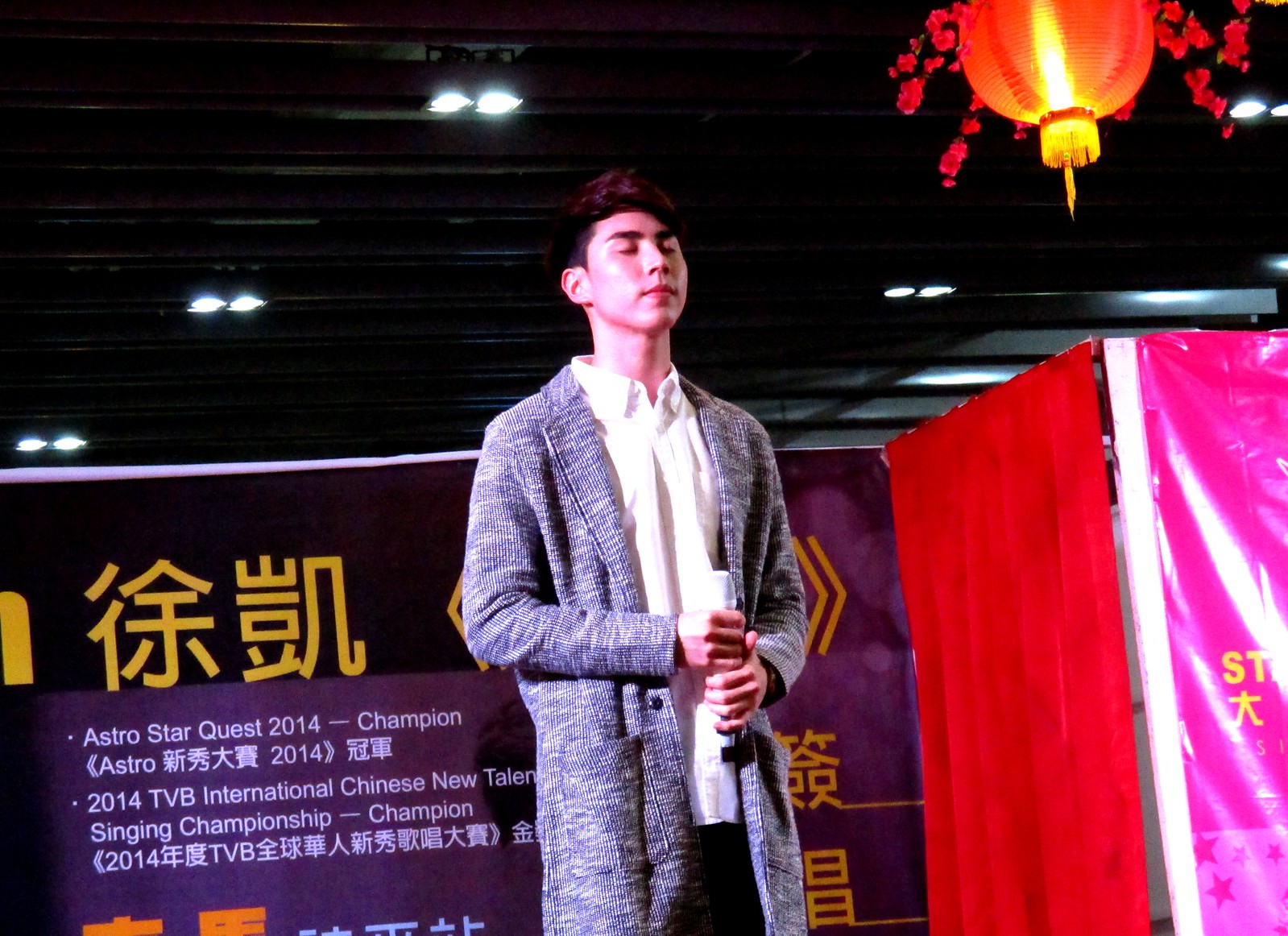The image captures a young Asian gentleman, standing on a podium with his eyes closed, seemingly preparing to sing in a competition. He is holding a microphone down by his waist, wearing a long gray-blue coat over a white collared shirt, and black pants. His short black hair is neatly combed to the side. Behind him, a banner in both Japanese characters and English reads "Astro Star Quest 2014 Champion" and "2014 TVB International Chinese New Talent Singing Championship Champion," indicating his victory in the event. The background is adorned with colorful curtains—yellow to his right and purple to his left—and a chandelier styled in Asian design. The ceiling is black, with bright lights shining down, creating a vivid and well-lit atmosphere. The image captures a moment of anticipation as the young man stands under the spotlight, about to perform.